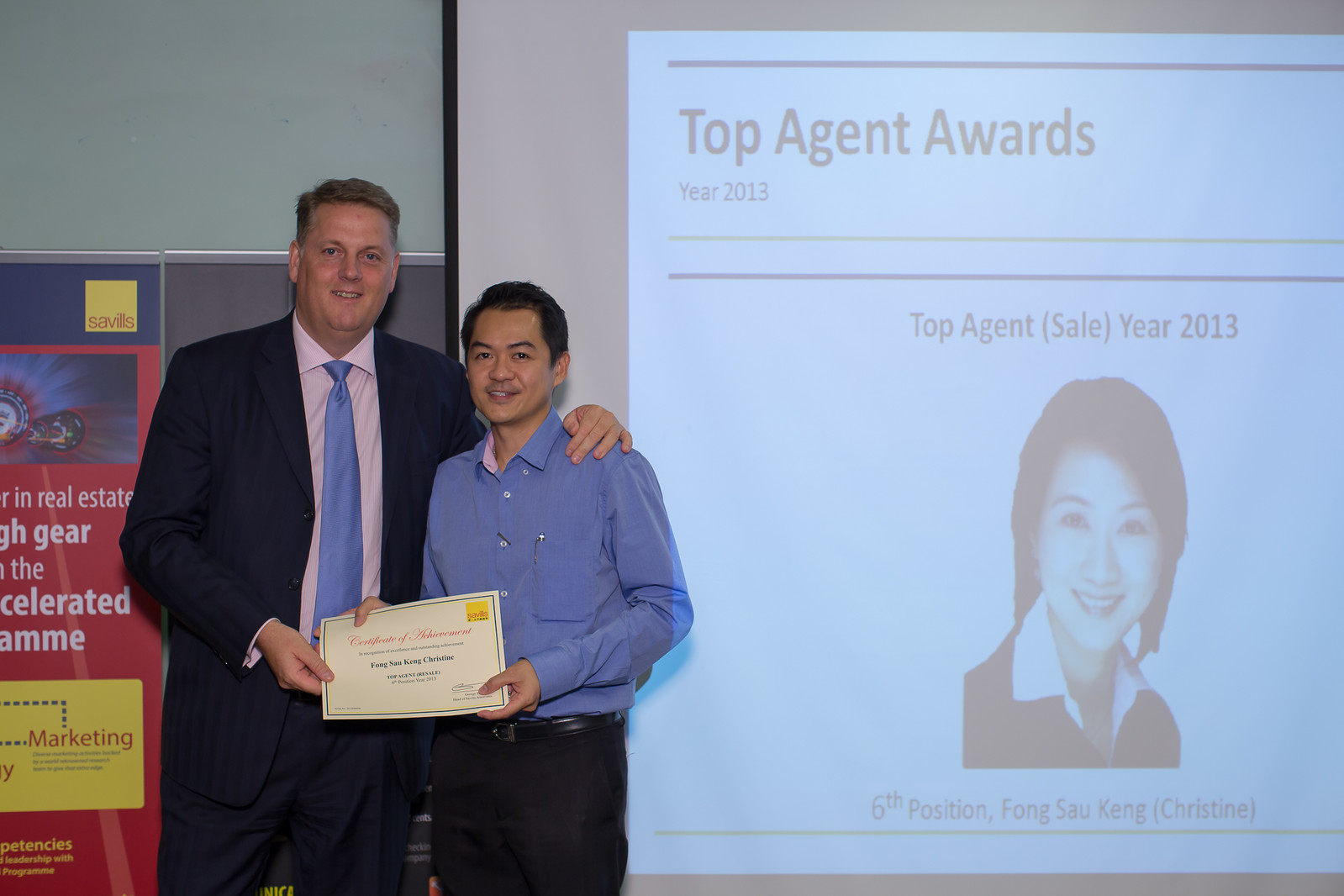The horizontally aligned rectangular image captures a moment during an award ceremony, featuring two men standing on the left side. The taller man, to the left, appears to be the presenter. He is dressed in a suit paired with a blue tie and a white collared button-down shirt. His short brown hair is neatly groomed, and he has his left arm around the shorter man beside him. The shorter man, presumably the award recipient, has short black hair and is wearing a long-sleeved button-down blue shirt. Both gentlemen are smiling slightly at the camera and are holding a "Certificate of Achievement" award, though the details of the award are not fully legible. Behind them is a large projector screen that reads "Top Agent Awards Year 2013" and displays a photograph of a woman with short, straight black hair. The screen indicates that she is the top agent in the sixth position for the year 2013, identified as Fong Sau Kang, also referred to as Christine. The background features a gray wall with a partial view of a red banner containing white text and a yellow rectangular section labeled "marketing," though the complete design is obscured by the left side of the picture.